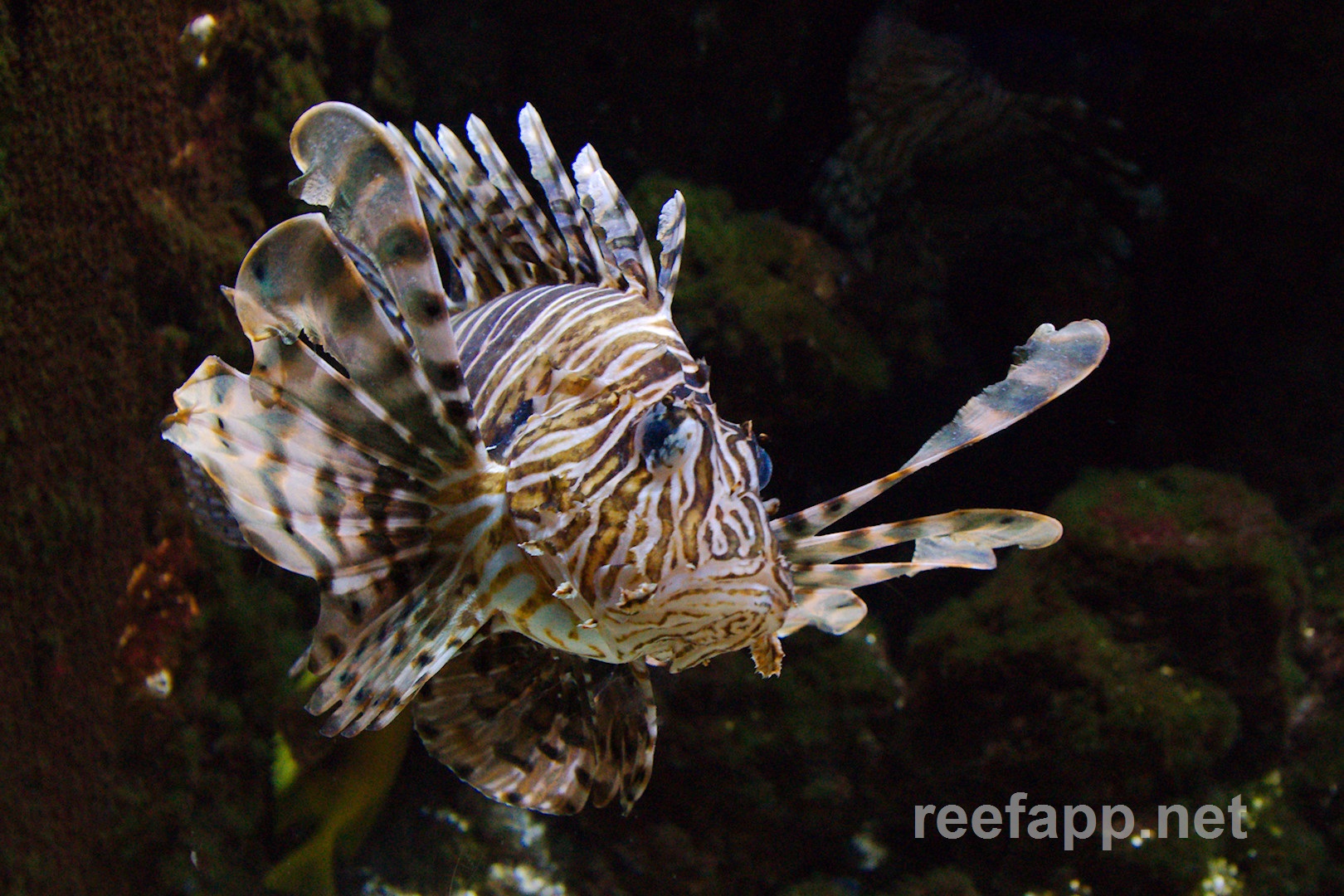The image is a close-up, detailed photograph of a lionfish swimming against a dark, undersea background featuring dark brown, corally rocks, and patches of green algae and moss. The lionfish is characterized by its distinctive, spiky fins that resemble a lion's mane, extending all along its back and sides. The fish exhibits a striking pattern of black, tan, and brown and yellowish-orange stripes covering its body and face, accentuated by large black eyes and a prominent mouth. A large, thick fin extends along the bottom of the fish, adding to its dramatic appearance. The scene is quietly intricate, with another faint, indistinct fish visible in the background at the top right. The caption "ReefApp.net" appears in white text at the bottom right corner of the image.